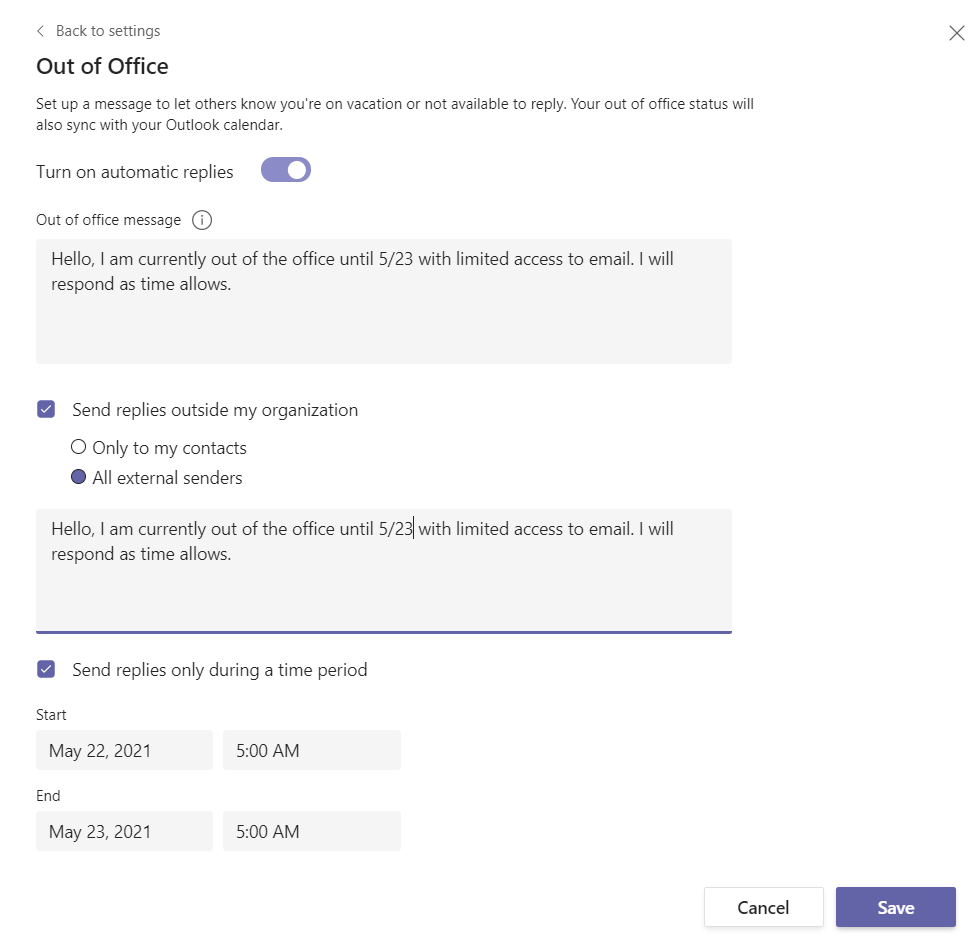The image depicts a user interface screen for configuring Out of Office settings. At the top, an arrow icon pointing left is labeled "Back to Settings." Below this, the heading reads "Out of Office." Beneath the heading is a paragraph of instructions followed by a toggle switch labeled "Turn on automatic replies," which is a purple button with a white circle on its right side.

Continuing down, there is a small circle with an eye icon, likely for informational purposes, followed by a gray square containing text. Below this gray square, there is a purple square with a checkmark and associated text. Next, there is an outlined gray circle with text beside it, adjacent to a purple circle with additional text. Another gray rectangle with more text is present below these circles.

Towards the bottom, a light purple line separates sections, and another purple square with a check mark appears with accompanying text. Following this, there is an input field within a white-gray rectangle for selecting a start date, and next to it, another light gray rectangle for choosing start time. The same format is repeated for end date and end time fields.

At the very bottom of the screen, there are two buttons: a white rectangle outlined in gray labeled "Cancel" and a purple rectangle labeled "Save."